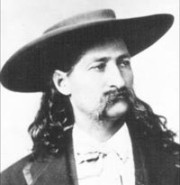This is a small, black-and-white photograph of Wild Bill Hickok, an iconic figure from the late 1800s. The image, which is frequently seen on historical and Wild West sites, is characterized by its simple yet striking features. Wild Bill is captured in a three-quarter view, looking to the left. He sports a long, dark handlebar mustache and long curly hair that falls past his shoulders. He is dressed in a black coat with gold trim and a white shirt, adorned with a subtle design on the collar. His distinctive cowboy hat, which features a flat top and low brim, sits securely on his head. The photograph, devoid of any background, focuses entirely on the upper portion of his body. Rendered in shades of black, gray, and white, this image exemplifies the style of the late 1800s and serves as a commonly recognized depiction of Wild Bill Hickok.